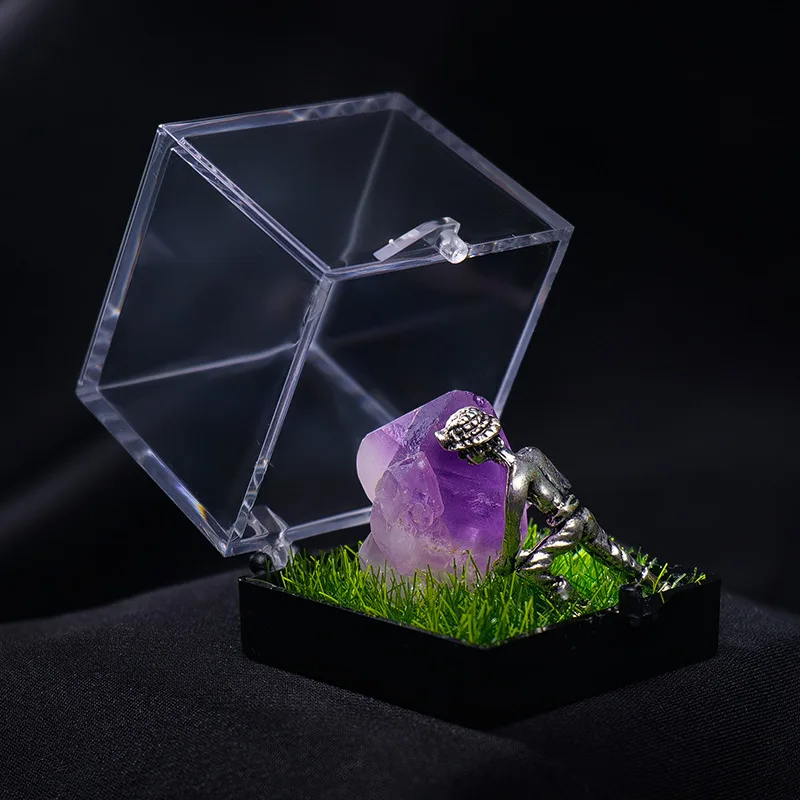The photograph captures a unique and detailed display set against a black fabric background, both on the surface and as a backdrop. The central object in this display is a clear plastic cubicle case, which has a black base and is opened along one side, showcasing its contents. The case features a latch on the front and hinges on the side, allowing for the transparent lid to be propped open. Inside, the primary focus is a sizable, stunning purple amethyst gemstone that transitions into a cream color under the light. This gemstone is nestled amid a patch of green grass, adding a natural touch to the setting. Adding to the intrigue, there is a small silver sculpture of a bare-chested figure wearing a hat and pants. The figure is positioned in a dynamic pose, facing away from the viewer, with its arms reaching down towards the gemstone and its feet braced against the edge of the box, suggesting an effort to lift or roll the much larger gemstone. The overall composition is striking and carefully arranged to draw attention to the intricate details of the gemstone and the whimsical silver figure.